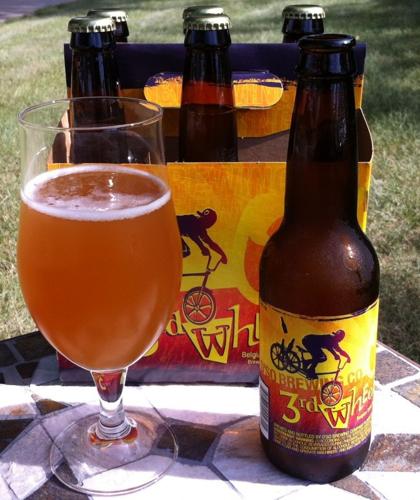The image depicts a rectangular photograph taken outdoors in daylight, capturing a scenic and detailed view of a six-pack of beer placed on the corner edge of a mosaic-style table made from various triangular and square-shaped stone chips in brown and white, all patched together with grout. In the clear foreground, there's an opened brown beer bottle with an artistic yellow, red, and orange label that features an image of a man with a backwards cap riding a tricycle; the tricycle has one wheel in the front, two at the back, and carries beer bottles in a basket. The label indicates it's from "Something Brewing Co." with the beer name "Third Wheel." Also on the table, to the left of the bottle, sits a clear glass filled with an amber liquid topped with a thin ring of foam. Behind the bottle and glass, a cardboard six-pack carrier with a handle holds five unopened bottles. The rest of the scene is complemented by lush green grass in the background, creating a serene and inviting outdoor atmosphere. The tablecloth beneath the six-pack and bottle features blue square designs with spikes emanating from each corner, making the setup both visually appealing and detailed.